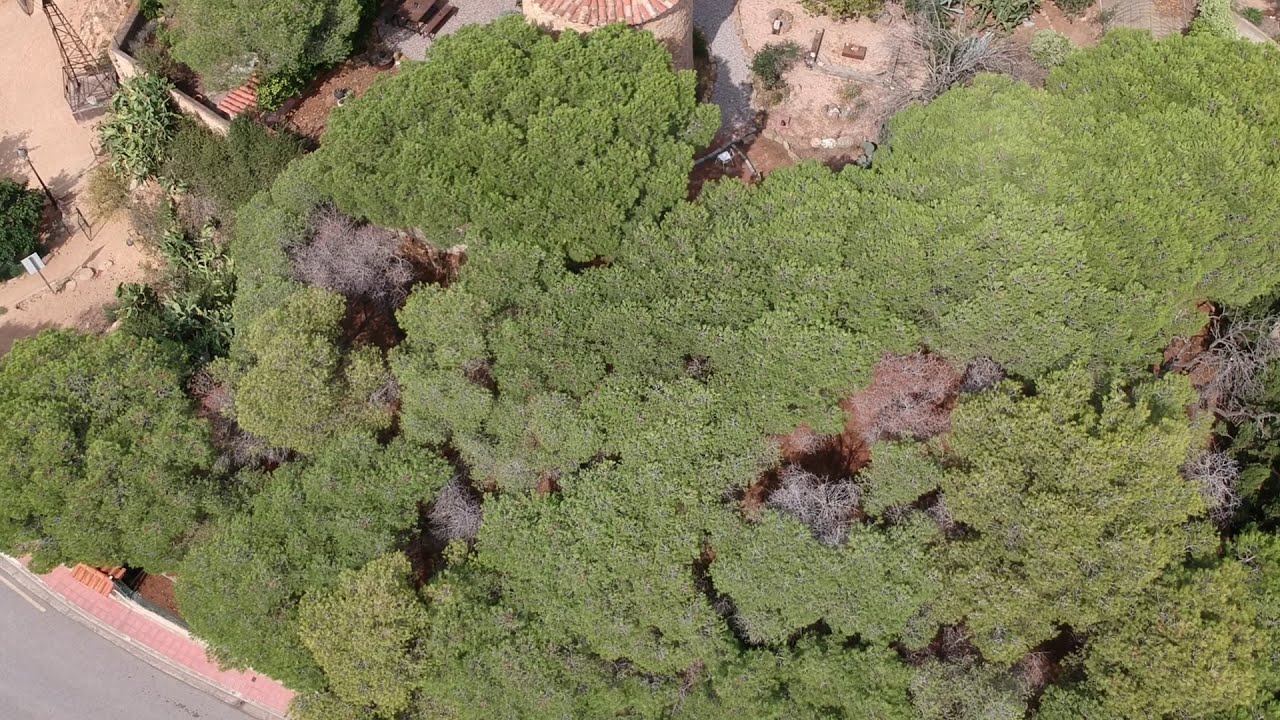In this vibrant aerial photograph taken on a sunny day, we are looking straight down on a dense canopy of lush, green trees, indicative of full summer. In contrast to the verdant foliage, a couple of trees stand bare, having already shed their leaves. In the lower left corner, a curved, black pavement road devoid of lane markings is visible, perhaps a single-lane road. Adjacent to it is a red brick walkway with a small bench along its side. The photograph captures more details in the upper left corner where brown sand or dirt patches are noticeable. A steel girder windmill, reminiscent of old-fashioned designs, stands prominently, and nearby streetlamp casts its presence over the scene. Additionally, a partially visible building with a cylindrical, stone structure crowned by a French tile roof adds architectural interest. A white sign, seen from its back, peeks into the frame from the center far left, while the consistent green of the tree canopy dominates the majority of the image.